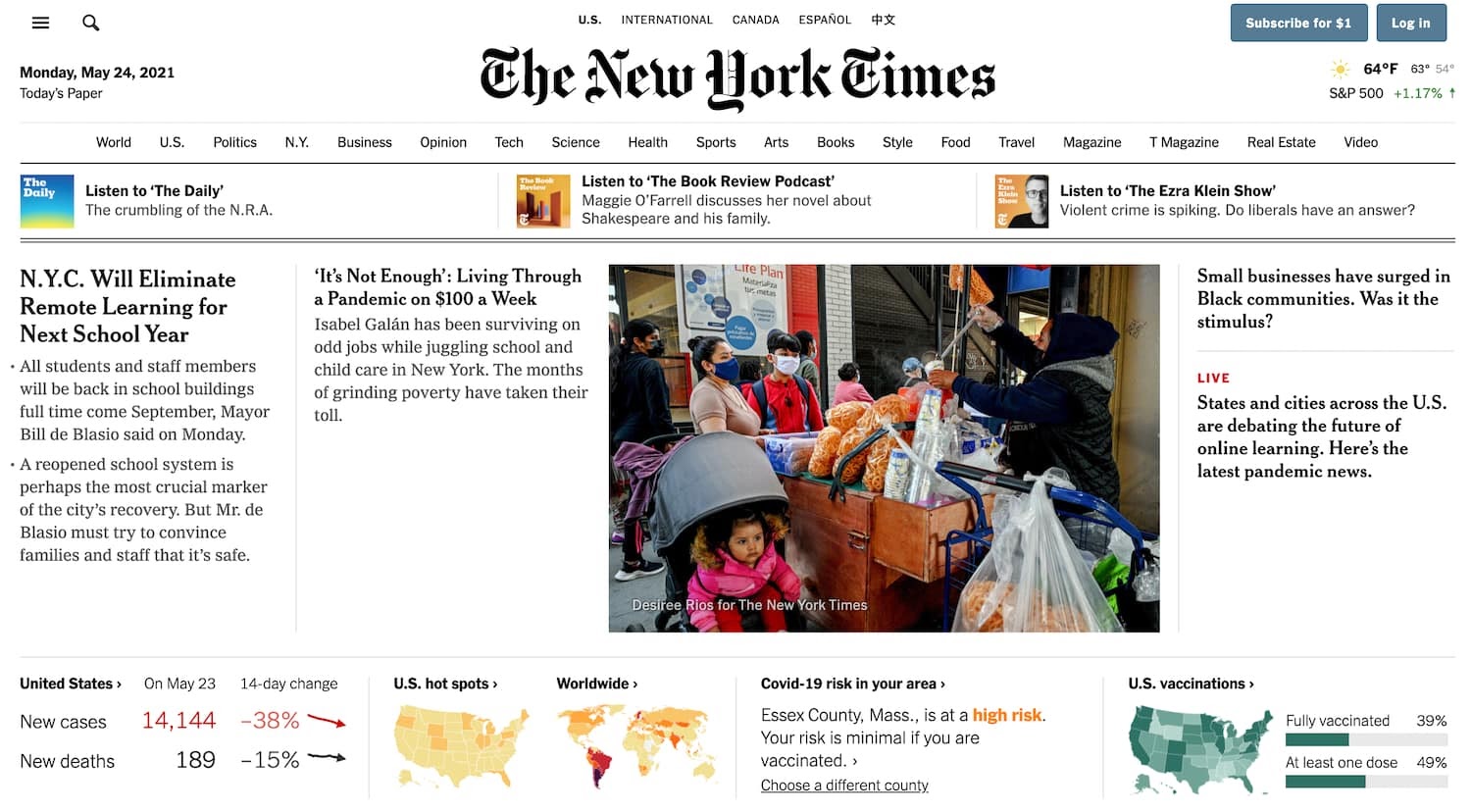This is a screenshot of the New York Times website displayed on a computer. The header prominently features the "New York Times" title in a large, elegant calligraphy-style font, centered at the top. On the left side of the screen, there is a hamburger menu icon and a search button. Below the header, the date "Monday, May 24th, 2021" is displayed, followed by a label for "Today's Paper." A horizontal navigation bar spans the width of the page, listing various topics such as "World," "U.S.," and "Politics."

Beneath this navigation bar, there is another section divided into three segments, each containing a small square image on the left and text encouraging the reader to listen to specific content on the right. Further down, a larger column displays the main news stories. On the left, a smaller headline announces "New York City Eliminates Remote Learning for Next School Year." To the right, a more prominent story, accompanied by an image, discusses the ongoing pandemic. At the bottom of the screenshot, a border presents COVID-19 statistics, providing an updated snapshot of the situation.